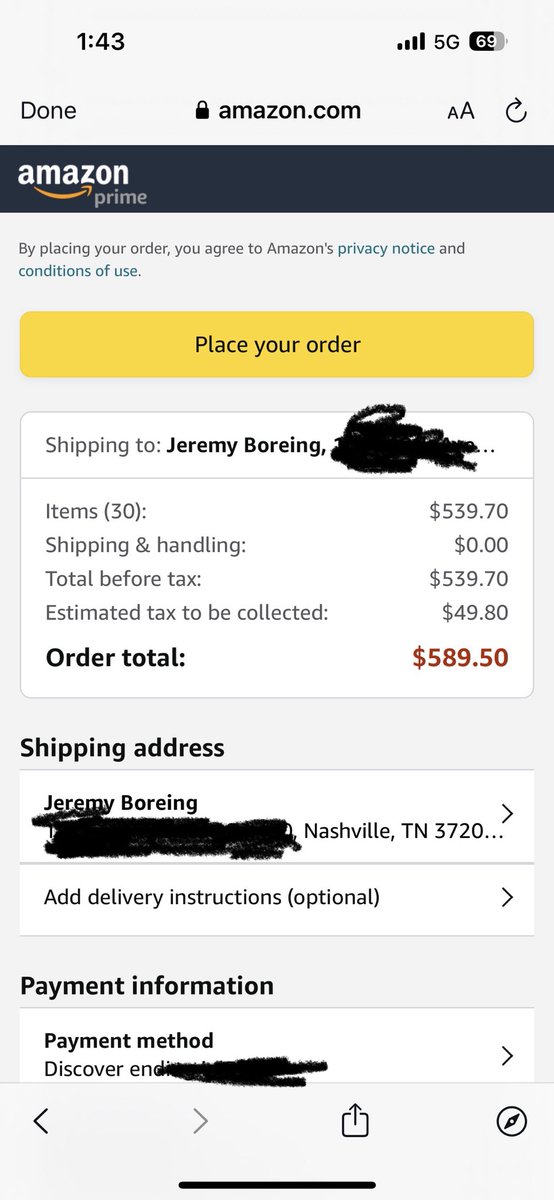A screenshot of a phone's display showing an Amazon order confirmation receipt. At the top of the screen, the phone status bar indicates the time as 1:43, full cellular service with four bars, 5G network, and a battery life of 69%. Below the status bar, the browser displays "Done" alongside "amazon.com" with a lock icon to indicate a secure connection, and options to adjust text size and an undo or back button.

A blue bar beneath this reads "Amazon Prime" featuring the Amazon logo with white lettering and the signature orange arrow from 'A' to 'Z', followed by 'Prime' in gray text. The main section starts with a notice: “By placing your order, you agree to Amazon's Privacy Notice and Conditions of Use,” with hyperlinks to the privacy notice and conditions of use.

A gold “Place your order” button is prominently displayed below the notice. Following this, the receipt details include:

- **Shipping to:** Jeremy Boring (with an "Edit" button next to the name).
- **Items:** $539.70.
- **Shipping and handling:** $0.00.
- **Total before tax:** $539.70.
- **Estimated tax to be collected:** $49.80.
- **Order total:** $589.50.
- **Shipping address:** Jeremy Boring, Nashville, Tennessee (with a forward arrow to expand details).

Beneath the address details is an option to "Add delivery instructions" marked as optional, followed by payment information:

- **Payment method:** Discover (last four digits obscured for privacy, with a forward arrow for more details).

Finally, at the bottom of the screenshot, there are navigation buttons for back, forward, download, and another icon that appears to be related to time management.